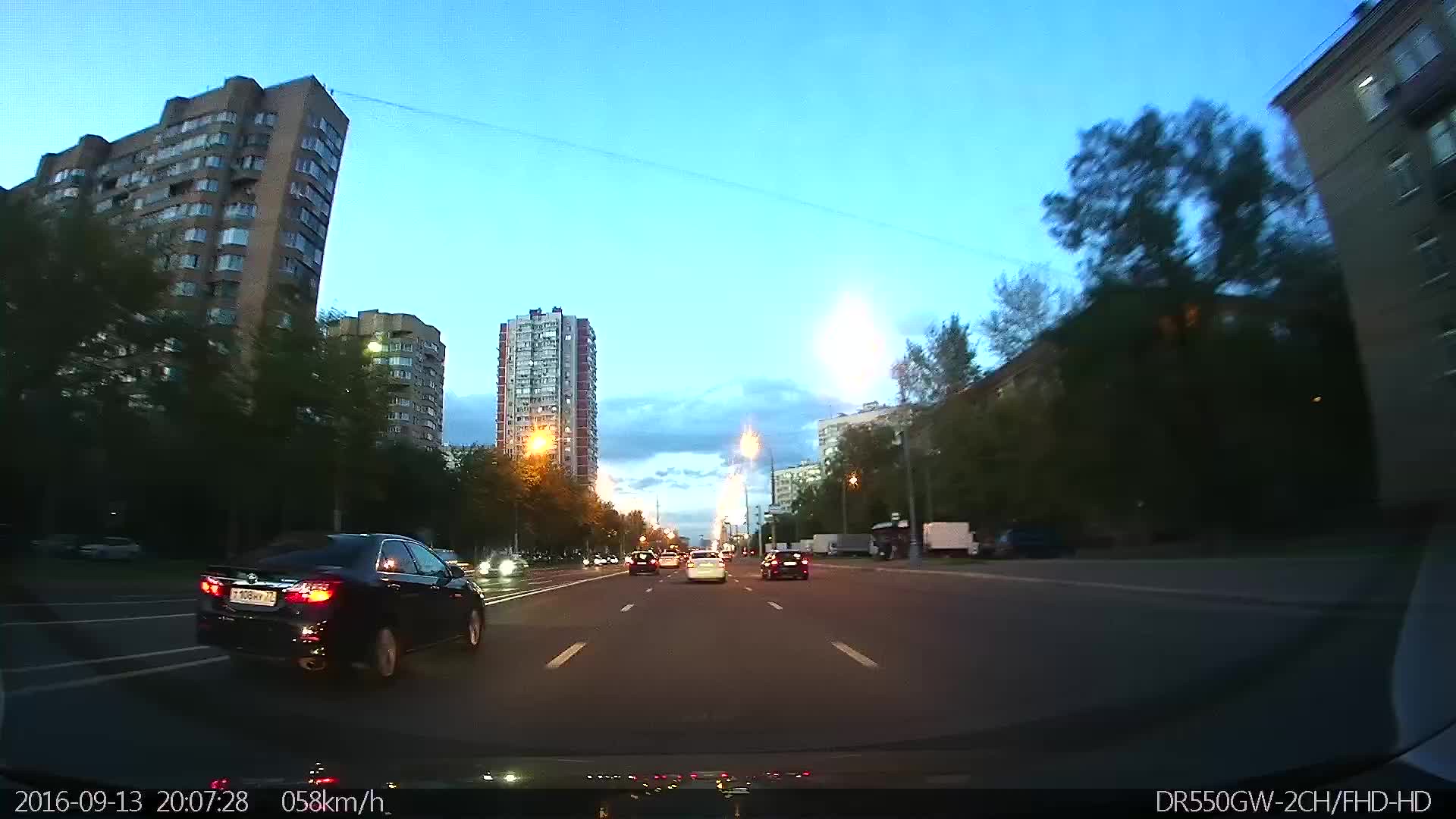This point-of-view photograph captures the scene of someone driving down a three-lane road during either dusk or dawn. To the left, three towering high-rise buildings dominate the skyline. In the same direction as the photographer's vehicle, a black car with its taillights illuminated can be seen in the left lane. Directly in front of the photographer's vehicle is a white car, flanked on both sides by two black vehicles. On the right-hand side of the road, a few streetlights are illuminated, casting a gentle glow over the scene. Behind the streetlights, trees are visible, adding a touch of nature to the urban environment.